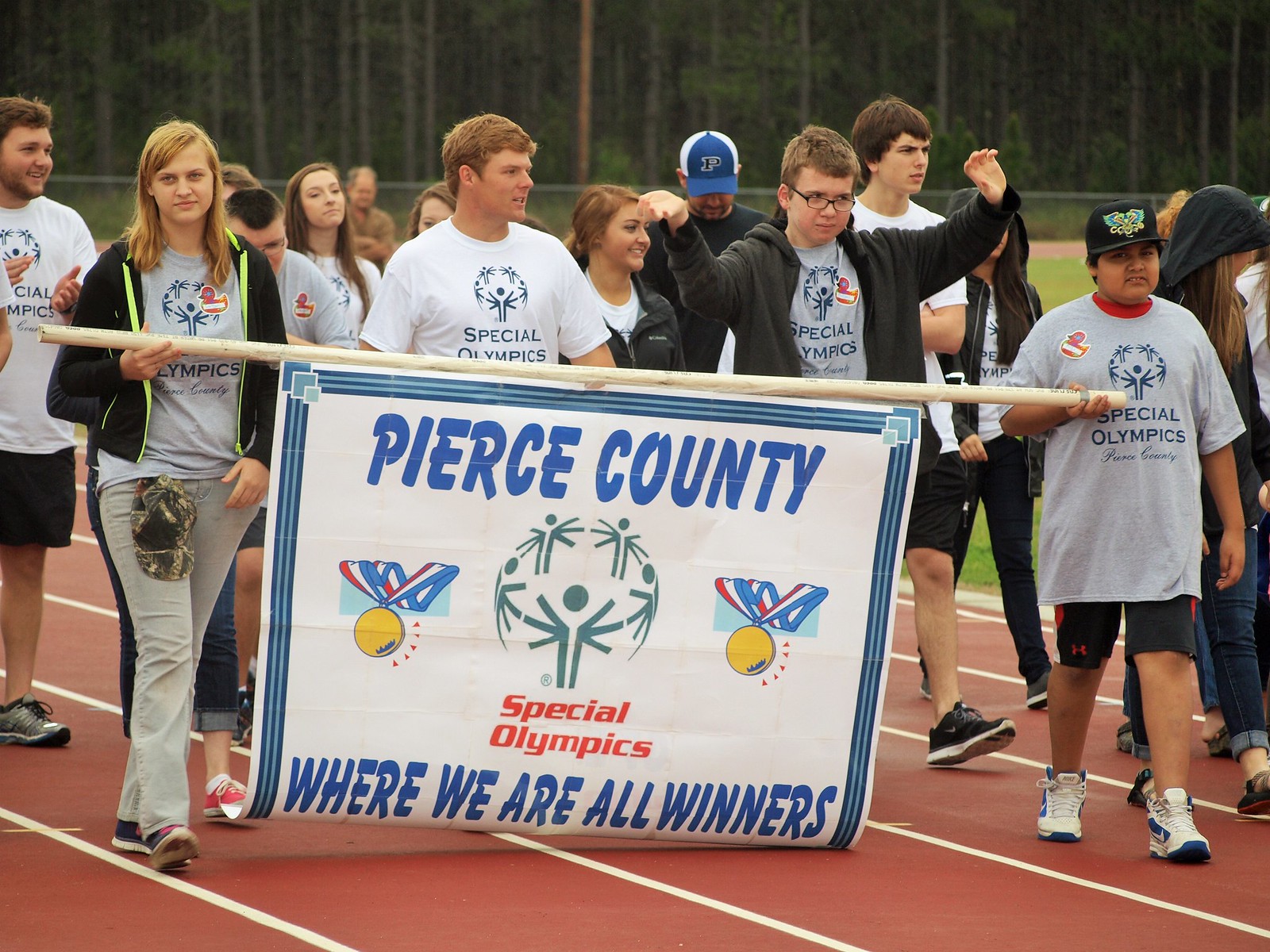In this image, a diverse group of people is walking together on a red track field, which features white lane markings. The participants, who appear to be of varying ages and likely include students, are part of the Special Olympics event hosted by Pierce County. Leading the group are a young girl on the left and a young boy on the right, both holding a yellow pole horizontally. Attached to the pole is a banner with blue text reading, "Pierce County Special Olympics, where we are all winners," and showcasing two gold medals. The participants are wearing Special Olympics t-shirts that range in color from gray to white. In the background, a chain-link fence stretches from left to right, beyond which stands a line of tall trees with green leaves and pine needles, contributing to the scenic setting of the event.